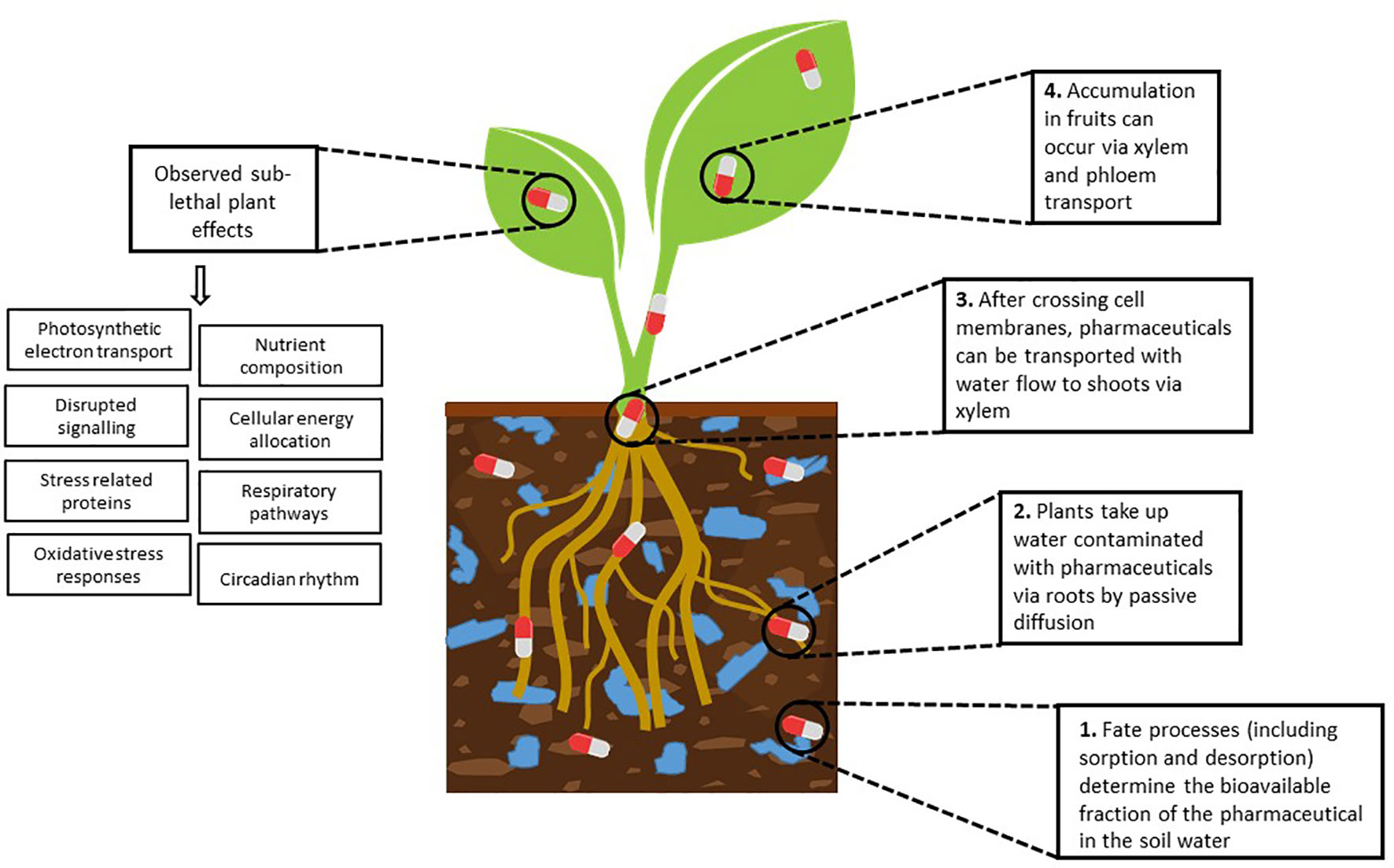This detailed illustration, reminiscent of an image from a scientific textbook, depicts a cross-sectional view of a plant showing both its above-ground and below-ground structures. The plant's green stem and leaves rise above the surface, while its tan-colored roots extend into the brownish soil below. The soil features blue markings, possibly indicating the presence of various nutrients or compounds.

Accompanying the visual are numerous annotations that elaborate on biological and chemical processes. To the left of the plant, there is a heading that reads, "Observe sub-lethal plant effects." Below this heading, two columns highlight processes involving photosynthetic electron transport among other detailed phenomena.

On the right side, numeric labels range from 4 at the top to 1 at the bottom, each within a box containing a specific description. The topmost box, labeled as number 4, explains that "accumulation in fruits can occur via xylem and phloem transport." The lowest box, numbered 1, states, "Fate processes, including sorption and desorption, determine the bioavailable fraction of the pharmaceutical in the soil water."

This thorough annotation provides a comprehensive understanding of how substances interact with plant systems, both at the molecular level and within the broader context of soil and plant physiology.